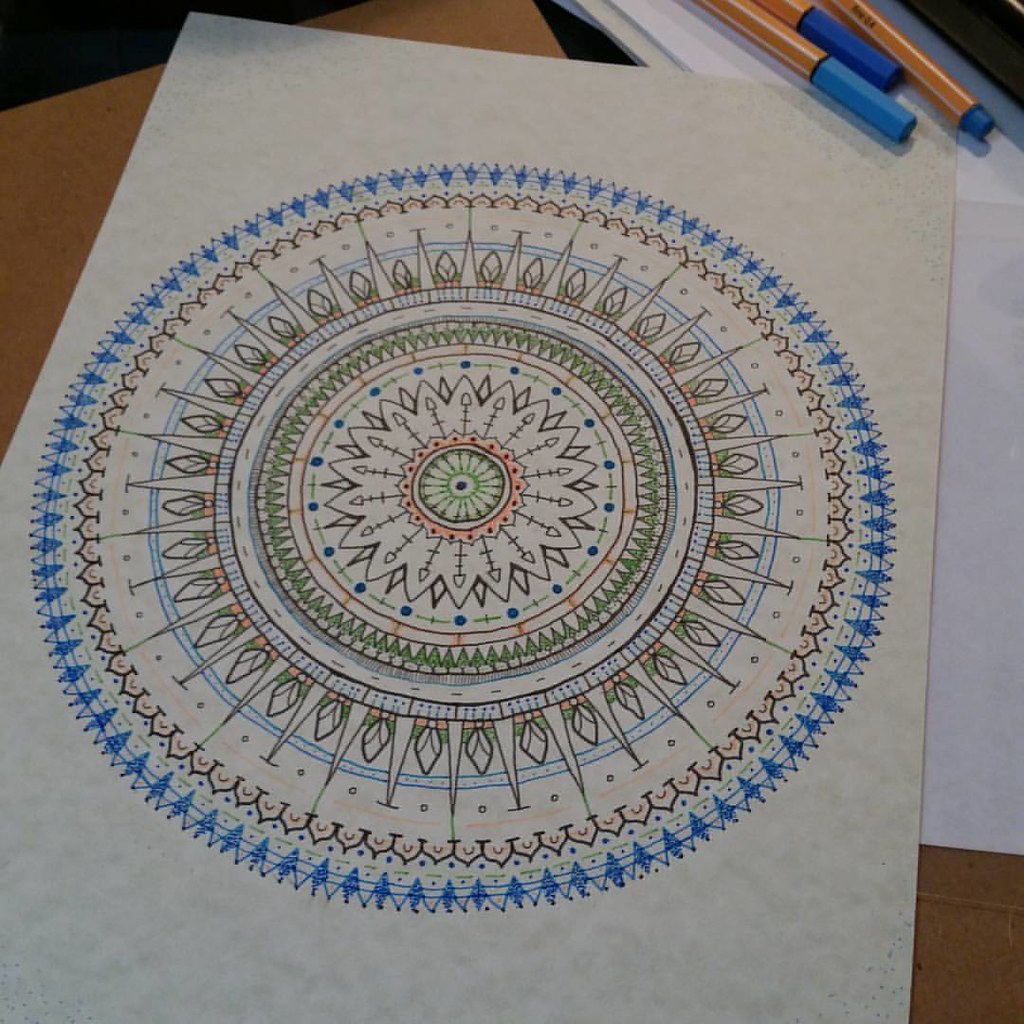The photograph captures an A4 sheet of sketch paper resting on a brown desk, accompanied by a blank white piece of paper situated to its right. The central focus of the artistic piece on the sketch paper is an ornate, mandala-like design consisting of intricate, concentric circles radiating outward from a central dot. The middle of the artwork features a green and white floral pattern, with the outer edges accented in blue. The mandala is detailed with patterns drawn in blue and black ink, and it is further colored in with red and green pencils. Above the artwork, there are ink pens, identifiable by their yellow bodies with white stripes, and colored tips and caps in shades of purple, dark blue, and light blue.